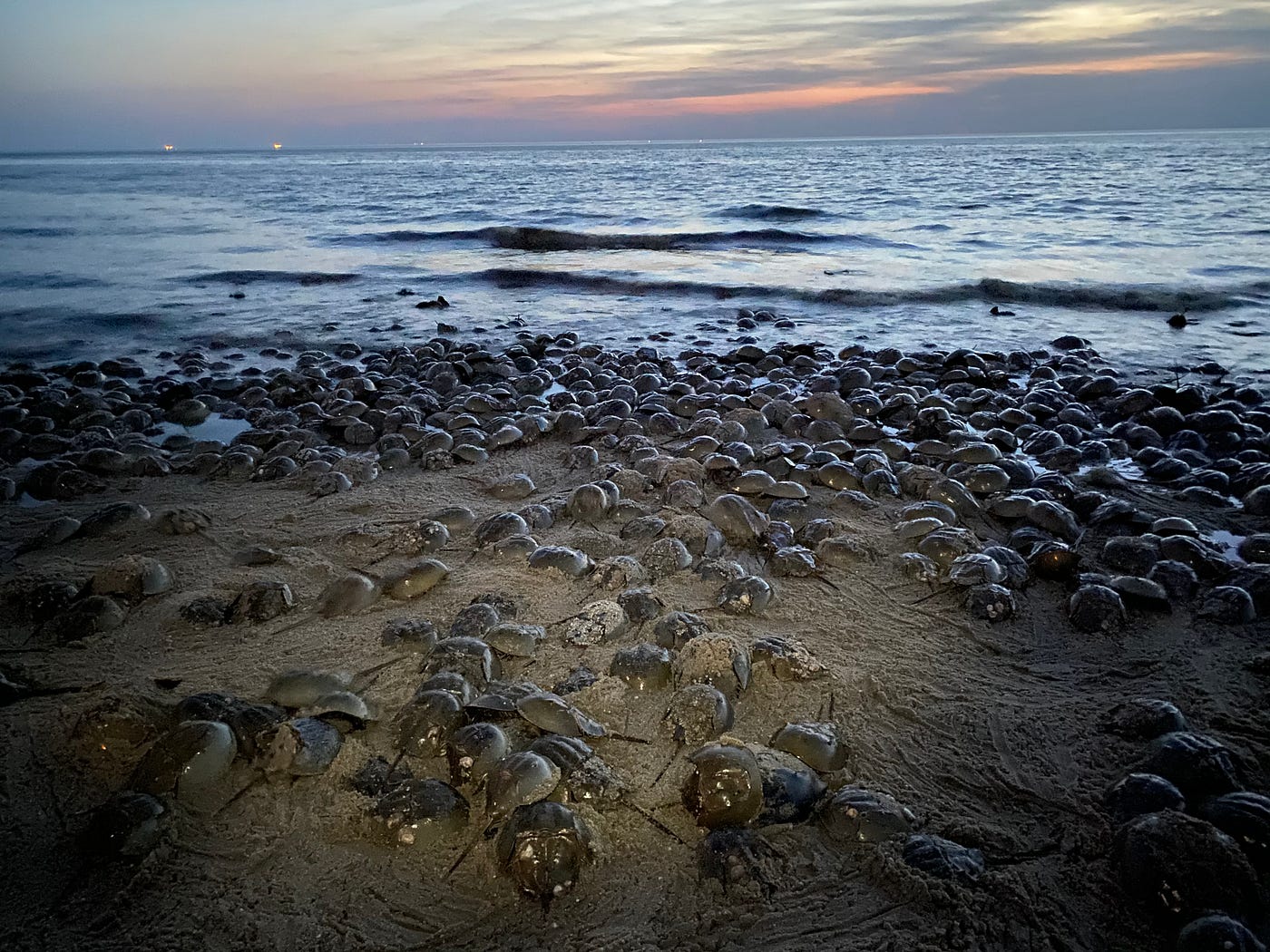The image captures a serene beach scene at twilight, where the sun has just set, casting a soft, warm glow of orange and pink that mingles with the purple and blue hues of the scattered clouds in the sky. The calm, dark blue ocean is softly lapping against the brown sand, with gentle waves barely disturbing the surface. Covering the sandy shore are thousands of horseshoe crabs, creating a surreal, almost otherworldly carpet. These crabs are densely packed, some stacked upon each other, forming an extensive, textured expanse. Many are making their way toward the water, while others are still partially buried in the sand or emerging from it. The sheer number of these green-shelled creatures moving en masse is striking, filling the scene with an extraordinary sense of life and movement against the tranquil backdrop of the dusky horizon.